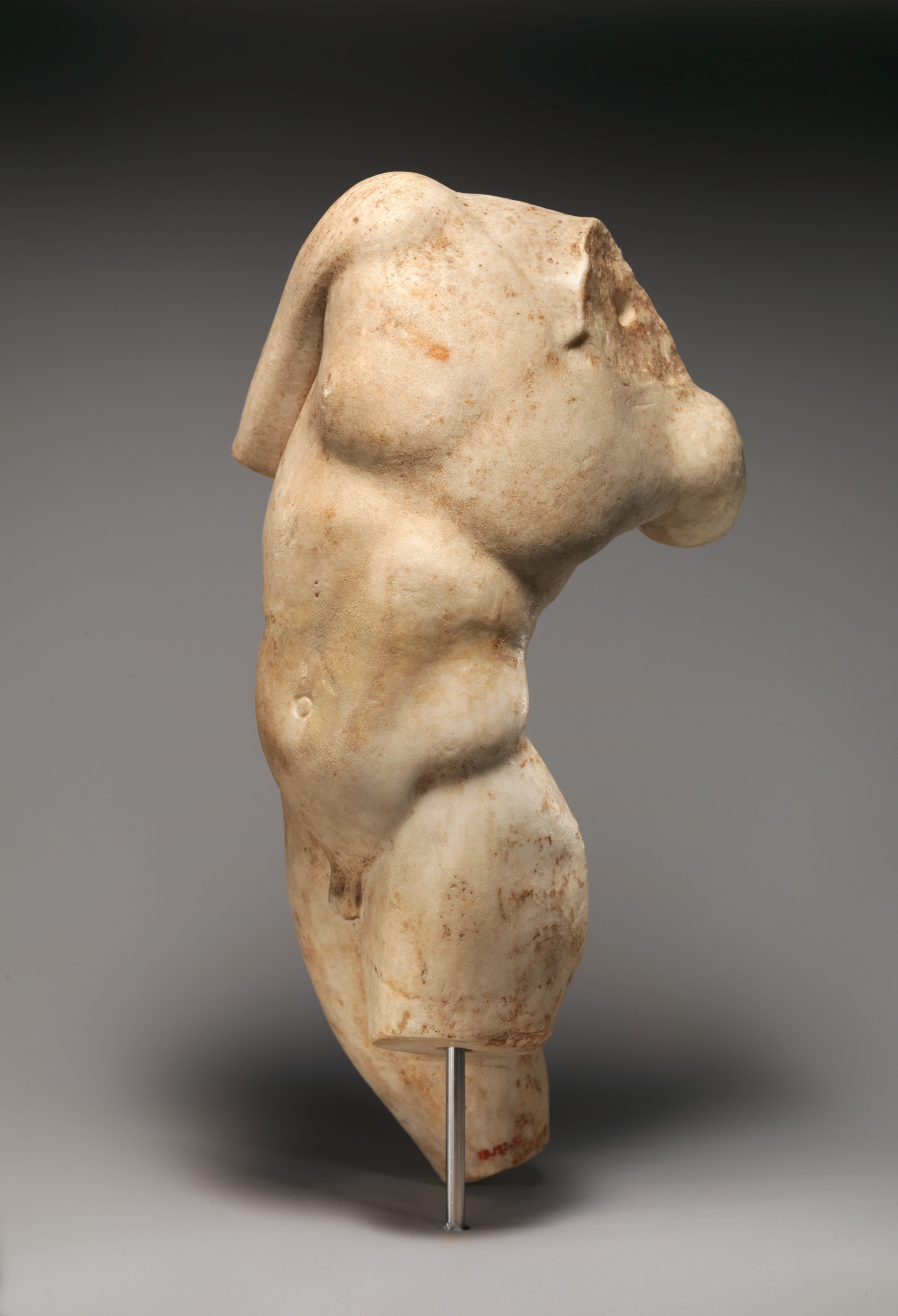The image showcases a detailed sculpture of a male torso cast in a material that appears to be some form of stone or possibly a hardened clay. The sculpture is predominantly white with sporadic brown specks, giving it a textured appearance. The figure is depicted from the chest down to the mid-thigh region, devoid of any clothing and positioned on a simple light gray surface that blends into a slightly darker gray background. This backdrop provides a neutral canvas that highlights the form and shadow of the sculpture.

The torso is contorted in a complex posture, with the chest turned to the left while the upper body arches back and to the right. The left arm is completely absent below the shoulder, and the right arm is severed just above the elbow, leaving only a portion of the upper arm. The head is missing, with jagged edges around the neck suggesting it may have been broken off.

The legs of the sculpture are asymmetrical in their truncation. The left leg is cut off mid-thigh, supported by a thin metal rod extending from the leg's center down to the base, providing stability. In contrast, the right leg is positioned behind the left and extends further down but still ends above the knee, not quite reaching the surface on which the sculpture stands. The overall ambiance of the image is well-lit, ensuring that the details and the intricate posture of the sculpture are distinctly visible.